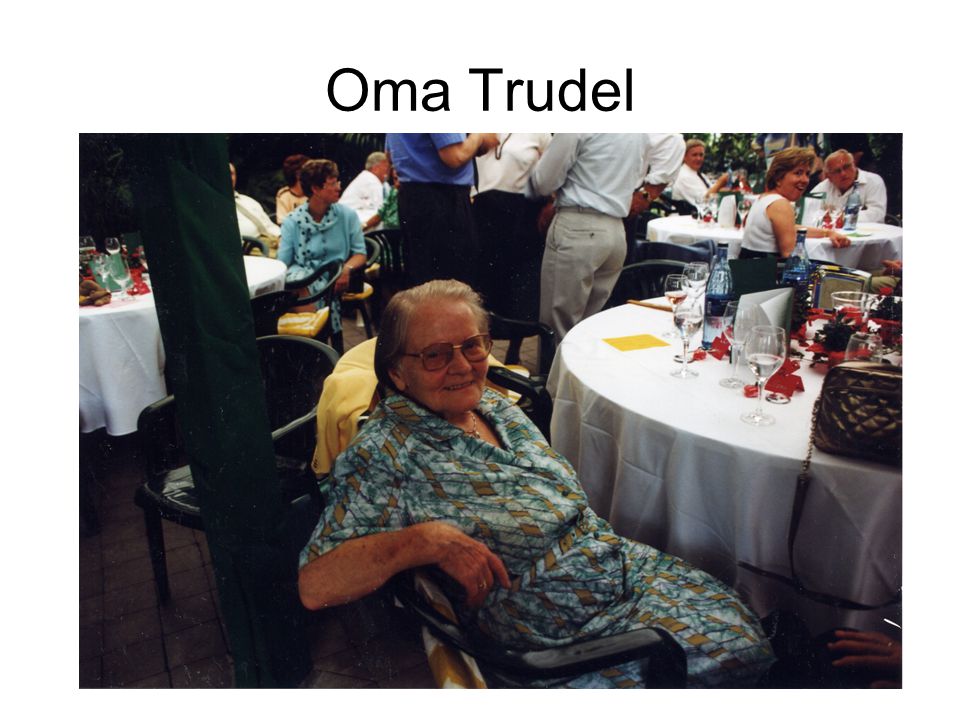The image depicts a lively indoor event, likely a catered party, reunion, or wedding, taking place in a spacious room with wooden floors. Round tables, adorned with white tablecloths, are scattered throughout the room. Each table has wine glasses and floral centerpieces for decoration. Guests, dressed in casual attire, are either seated in black resin lawn-style chairs with arms or standing around engaging in conversation.

At the forefront of the image sits an elderly woman, identified by the text at the top of the image as "Oma Trudel." The text, written in black font on a white border, suggests the image might be part of a slideshow presentation. Oma Trudel, dressed in a light blue and gold patterned dress, is captured in a relaxed pose with her arm draped over the back of her chair. She gazes directly at the camera through her yellow-tinted, wire-framed glasses. Beside her on the round table is a gold-toned, soft purse, amidst scattered rose petals. The image, with its rich array of colors and detail, highlights both the celebratory atmosphere and the warmth of the gathering.